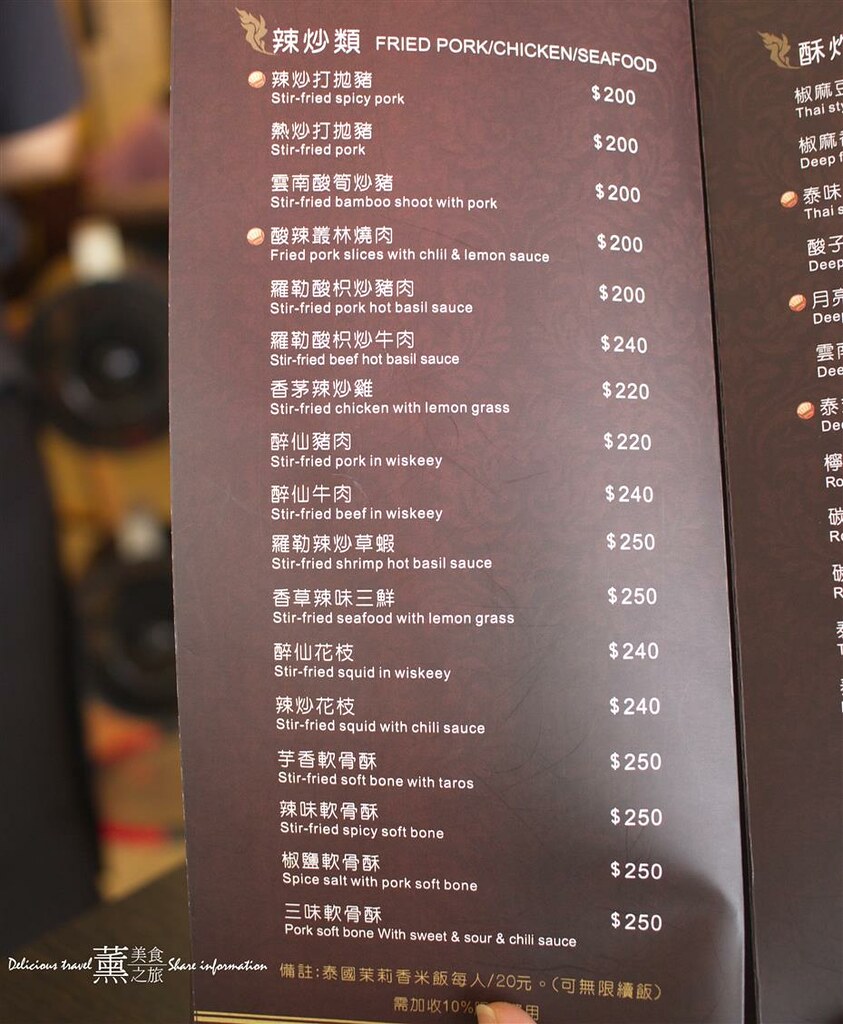This detailed photograph captures the essence of an authentic dining experience by showcasing a restaurant menu held open by a person, revealing its left page. The menu is presented in a rich deep red background adorned with a delicate filigree pattern. At the top, bold text reads "Fried Pork / Chicken / Seafood" accompanied by Chinese or Japanese characters, emphasizing the menu's cultural authenticity.

The listed items include:

- Stir-fried Spicy Pork - $200
- Stir-fried Pork - $200
- Stir-fried Bamboo Shoot with Pork - $200
- Fried Pork Slices with Chili and Lemon Sauce - $200
- Stir-fried Pork Hot Basil Sauce - $200
- Stir-fried Beef Hot Basil Sauce - $240
- Stir-fried Chicken with Lemongrass - $220
- Stir-fried Pork and Whiskey - $220
- Stir-fried Beef and Whiskey - $240
- Stir-fried Shrimp Hot Basil Sauce - $250
- Stir-fried Seafood with Lemongrass - $250
- Stir-fried Squid and Whiskey - $240
- Stir-fried Squid with Chili Sauce - $240
- Stir-fried Soft Bone with Taros - $250
- Stir-fried Spicy Soft Bone - $250
- Spiced Salt with Pork Soft Bone - $250
- Pork Soft Bone with Sweet and Sour and Chili Sauce - $250

Each dish name is meticulously paired with corresponding Chinese or Japanese characters, further emphasizing the menu's cultural roots and authenticity. A faint outline of a person's thumb is visible at the bottom of the image, holding the menu open. The blurred background hints at the ambiance of the restaurant, revealing indistinct shapes including two black round objects and a shadowy figure in a pink shirt, giving a sense of the bustling environment.